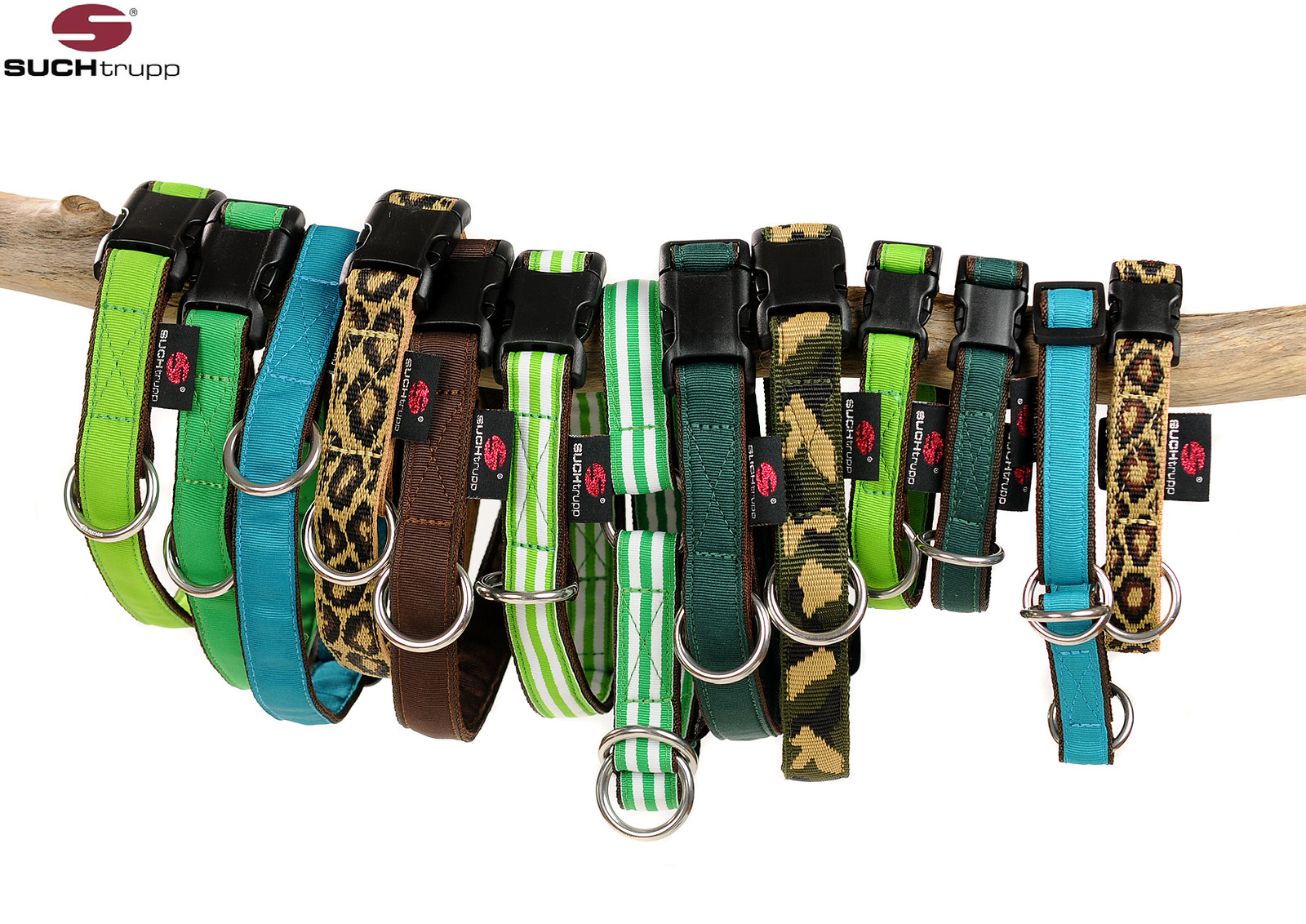This is a promotional photograph featuring a series of 13 small dog collars, neatly arranged on a light brown wooden branch against a white background. In the top right corner of the image, the brand name "Suchtrupp" is displayed with a distinctive maroon logo featuring a stylized "S". The collars are aligned one after the other, showcasing a variety of vibrant colors and patterns, each with black buckles and silver key rings.

From left to right, the collars include:
1. Bright lime green with brown borders
2. Forest green with brown borders
3. Light turquoise blue with brown borders
4. Cheetah print
5. Solid brown
6. White with lime green vertical stripes
7. Forest green with white vertical stripes
8. Dark green with brown borders
9. Camo style
10. Two smaller collars: one with lime green and dark blue patterns, both with brown borders
11. Bright blue with brown borders
12. Another cheetah print style

Each collar is meticulously designed, demonstrating the brand’s attention to detail and diverse style range.